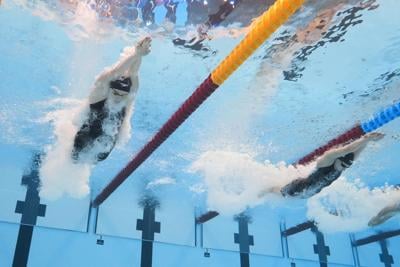This photograph captures an underwater scene in a swimming pool, likely during a competition or training session. The light blue water reveals the tiled pool floor, marked with alternating white, gray, and black squares, which guide swimmers from their dive start to their lanes. Floating lane dividers, colored in combinations of burgundy and yellow, as well as burgundy and blue, run parallel beneath the surface, segmenting the swimmer's paths.

Three swimmers dominate the scene. The swimmer on the left is fully visible, propelling towards the viewer with a black tank-style swimsuit, black goggles, and a black swim cap. Their hands are outstretched in a streamlined position above their head, breaking the water with vigorous kicks, producing clouds of white bubbles behind them. Parallel to this swimmer in an adjacent lane follows another, similarly attired and positioned. Only the legs of a third swimmer, visible in the lower right corner, hint at their presence outside the main frame.

Above the water, the blurred colors and reflections suggest either an audience or surrounding structures, adding context to the energetic motion captured below. The overall composition, enriched by the contrasting lane dividers and dynamic bubbles, emphasizes the powerful and synchronized start of these athletes in their aquatic environment.